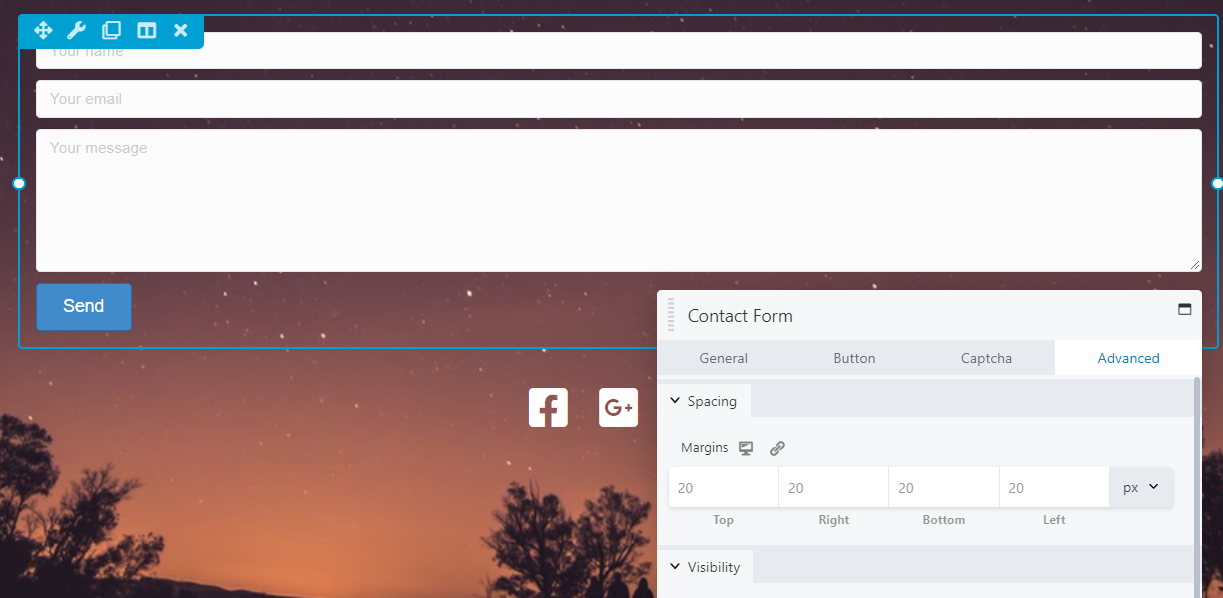The image showcases a webpage with a visually striking background of a reddish-orange night sky scattered with small stars. The silhouettes of tree branches are faintly visible at the bottom, adding depth to the scene. In the upper right corner of the webpage, a blue rectangular box contains various icons, including a wrench and an 'X'. 

Beneath this blue box, there is a long white rectangular field labeled "your name," followed by another similar field labeled "your email." Below the email field, a significantly larger white rectangular box—approximately five to six times the height of the previous fields—contains the text "your message." Underneath this large box, there is a small blue rectangular button with the word "send" displayed in white text.

On the far right side of the page, there is a contact form section with a gray background. This section is divided into several categories: "general," "button," "captcha," and "advanced." Below these categories are options for "spacing" and "margins," each listed with the number 20 for the top, right, bottom, and left margins respectively.